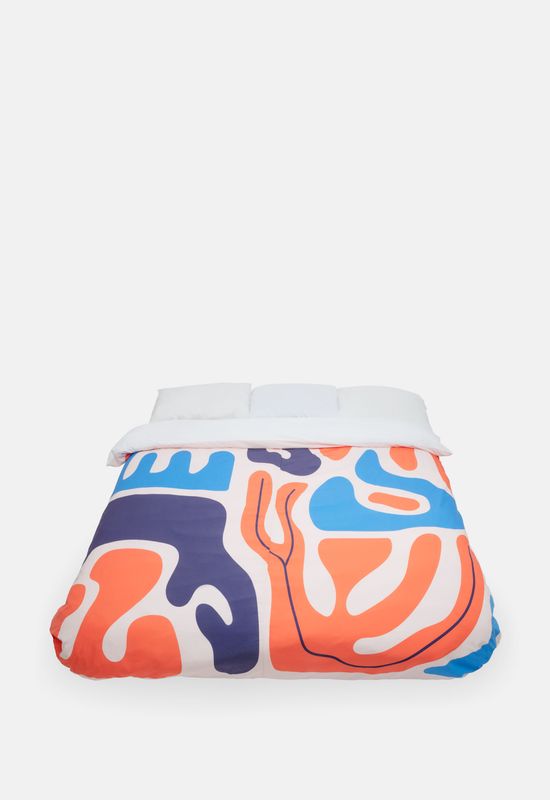This photograph features a simple mattress, possibly a queen or king-sized air mattress, laying on a stark, off-white floor. The bed is topped with a comforter that boasts an abstract art design. The comforter has a white background adorned with an array of irregular, swirling shapes in vibrant colors, including light blue, dark blue, orange, and purple. Some shapes have black lines that resemble coral or melted patterns, giving a dynamic visual effect. The comforter's top edge is folded down, revealing the white underside and three shiny white pillows laid end-to-end across the head of the mattress. The photograph is taken from above, about four feet away, providing a clear top view of the entire bed setup against the minimalist backdrop.